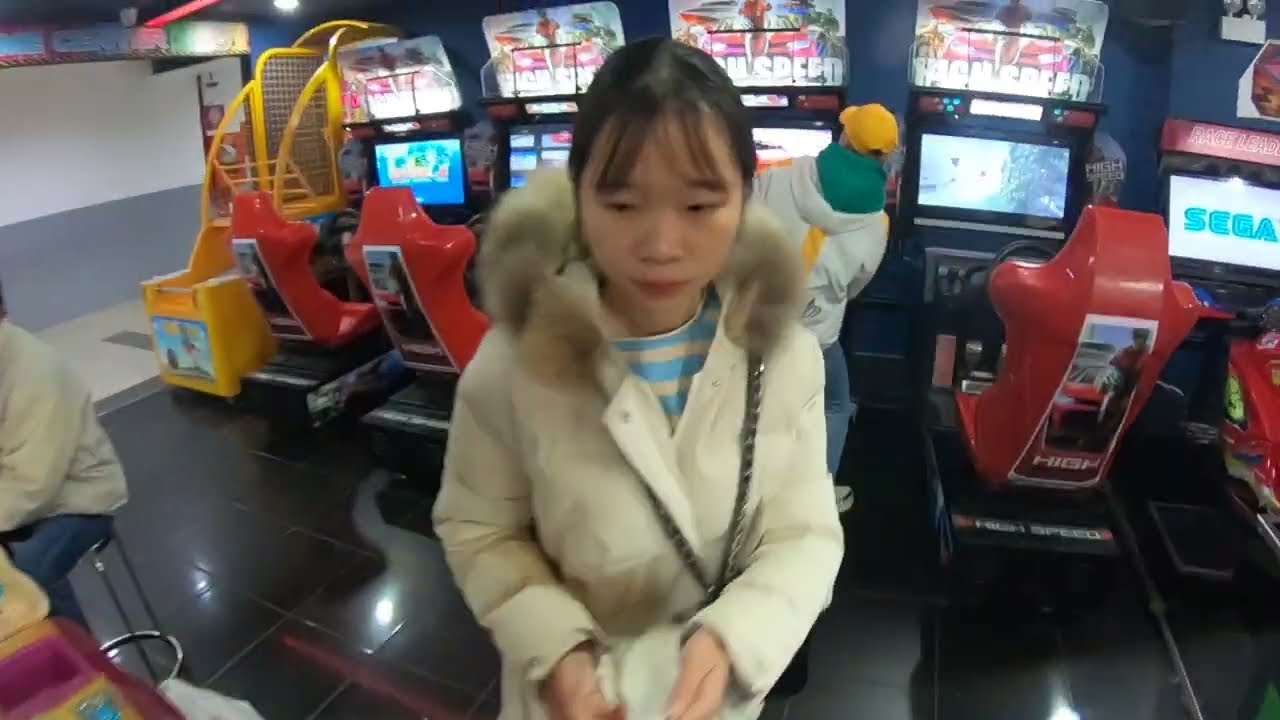In the heart of an arcade hall bustling with activity, an Asian woman, possibly of Korean or Chinese descent, stands as the focal point of the image. She has black hair and wears a cream-colored coat with a fur-lined hood, under which she sports a blue and cream-striped shirt. Her attention seems fixed on something ahead as she gazes downward, her hand delicately holding a small purse slung over her shoulder. The arcade scene around her is vibrant, with numerous driving simulation video game machines featuring seats and steering wheels. A man in the background dons a white hoodie and a yellow baseball cap while engrossed in a game, and a woman sits on a barstool to the left, probably engaged in another video game. The shiny, black-tiled floor reflects the bright overhead lights, and a sign bearing the word "SEGA" is visible in the distance, adding to the typical ambiance of an entertainment-filled arcade hall.